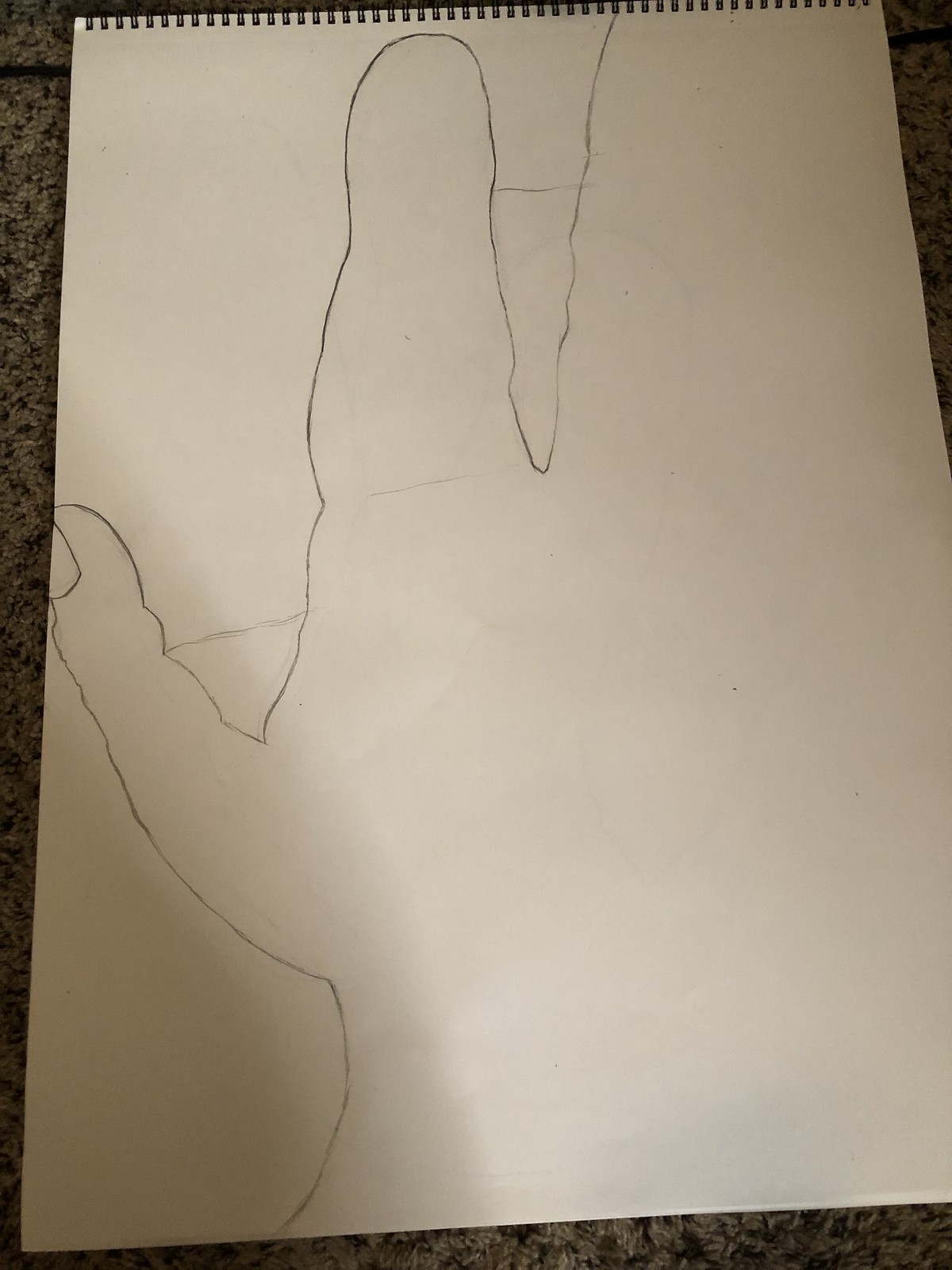The image showcases a dark gray and black speckled stone countertop, possibly marble, with various slivers of it visible around the edges. Atop this countertop lies a large artist's pad with black spiral binding along the top edge. The pages of the pad are rectangular and plain white. The featured page shows an unfinished pencil sketch of a hand, suggesting a right hand with an outstretched thumb and partially drawn index and middle fingers. The thumb nail is distinctly drawn, adding detail to the naive, almost childlike style of the sketch. The proportions of the hand are exaggerated, giving the appearance of an alien or deformed hand, particularly evident with the unusually large index finger. A light gray shadow is cast on the bottom left corner of the page, possibly from an object or person just out of frame.